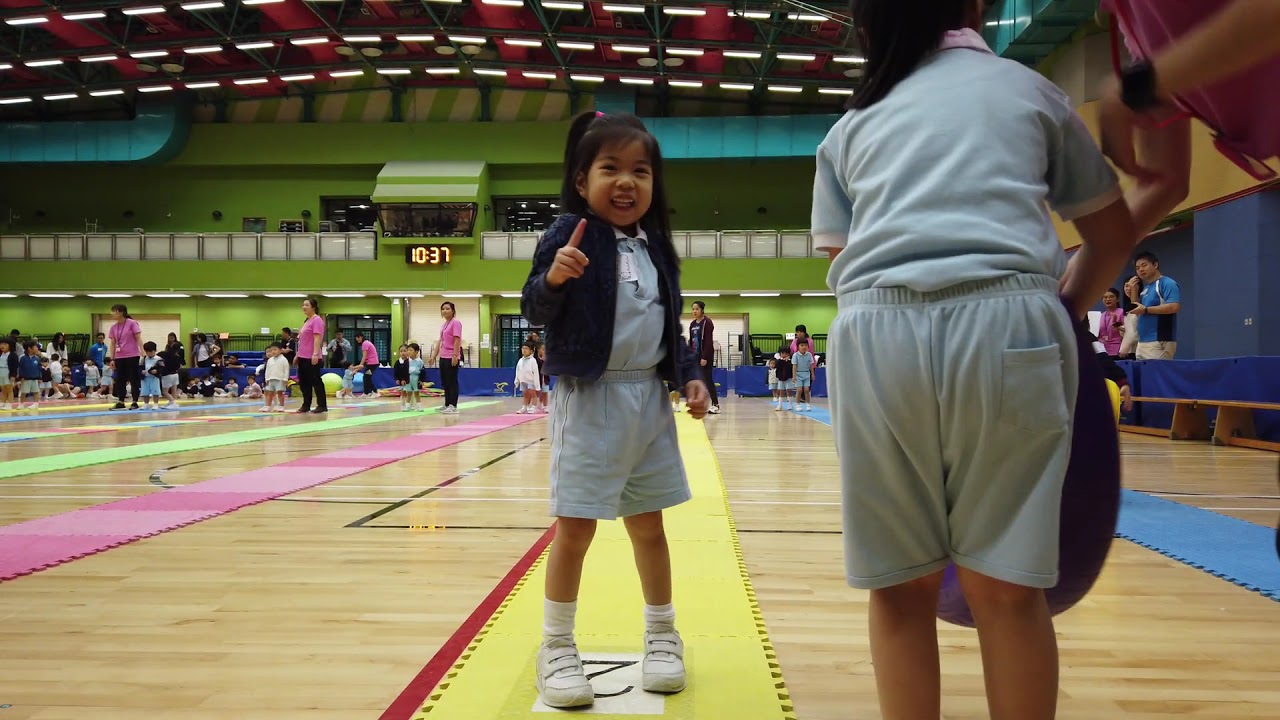In the bustling gymnasium with walls painted lime green, the wooden floor is covered with wide, colorful strips arranged as lanes — in green, pink, yellow, and blue, each about a foot and a half to two feet in width and separated by approximately four feet. The vibrant scene features numerous adults in pink t-shirts standing amidst the lanes, potentially overseeing a playful event. Center stage is a small Asian girl, no older than six or seven, with brown skin and black hair styled into a side ponytail. She stands confidently on a yellow lane marked with the number two, wearing light blue shorts and a matching t-shirt, and a navy blue jacket paired with white shoes. Her right index finger is pointed up, her face scrunched in a cheerful smile, looking directly at the camera and seemingly proclaiming herself as number one. To her right, a slightly taller child in a similar light blue outfit faces away, adding to the lively dynamic of the scene. In the background, perched above the activity, a timer reads 10:37, hinting at the organized, timed nature of the event.